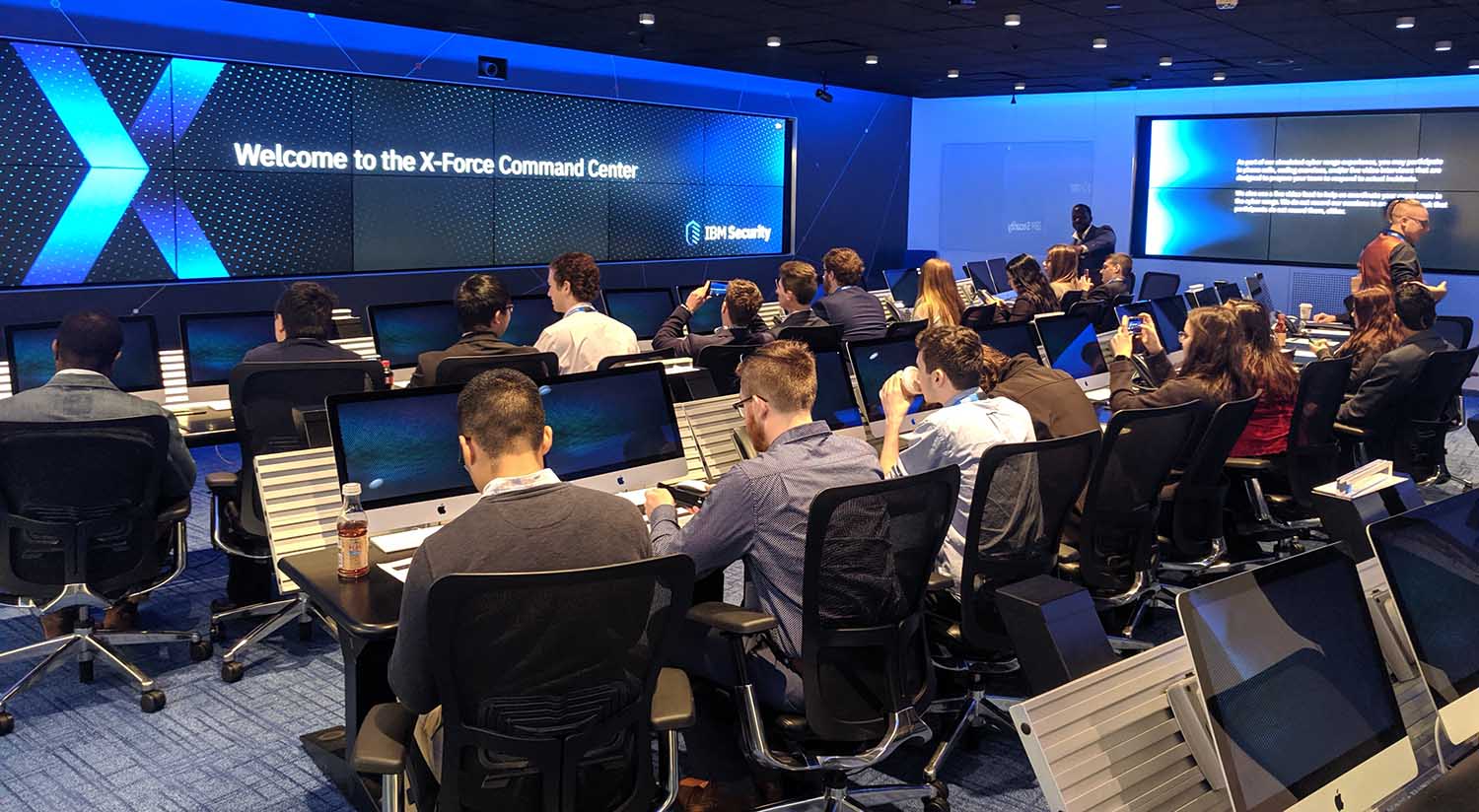The image is a detailed photograph of a high-tech command center, identified as the "X-Force Command Center". The room features three long black tables, each lined with Apple-branded Mac computers and keyboards, with people seated on one side in large black mesh office chairs. The middle table has eight individuals, each focused on their computer screens. Behind them and to the front, the setup is similar, indicating a highly organized environment. The walls of the room are painted blue, adorned with large TV screens composed of smaller units to form larger displays. Prominently displayed on the back wall is a message reading "Welcome to the X-Force Command Center" in blue and white letters, and a separate screen to the right shows "IBM Security" among other unreadable text. The ceiling is a black drop-down design with round white lights embedded. The overall blue color scheme and advanced tech setup emphasize the command center's immersive and professional atmosphere.